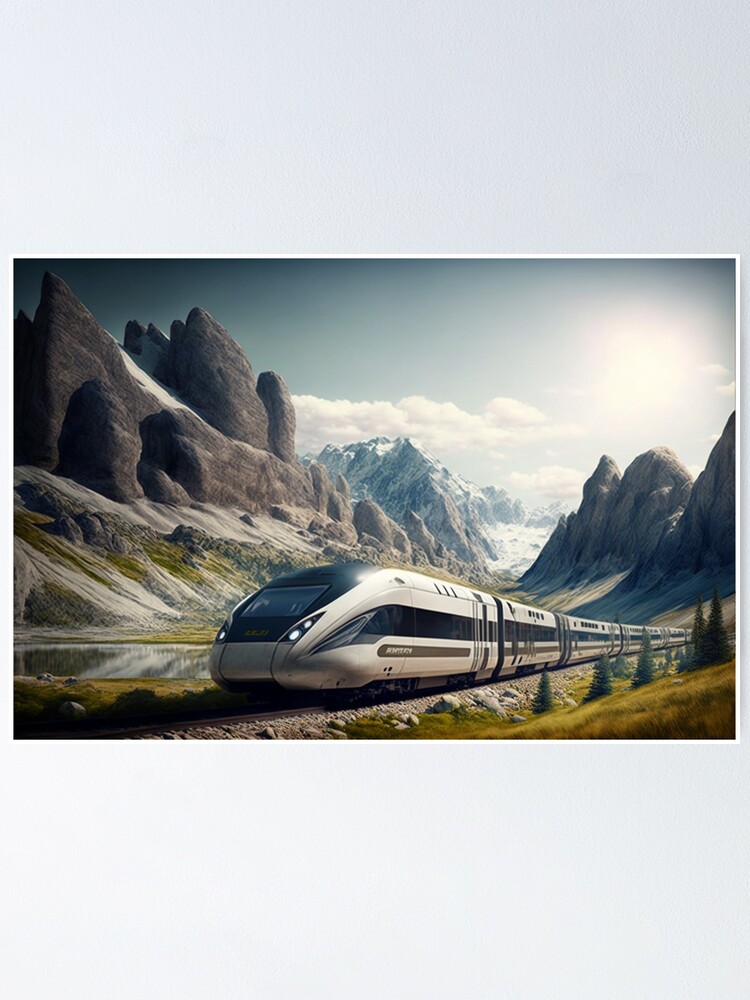This detailed image, which might be computer-generated or a photograph, showcases a sleek modern bullet train prominently positioned in the foreground. The metallic silver train, with its defining black stripe down the middle, starts near the left side of the image and trails off into the distance towards the right corner. The train, including the main power vehicle at the front with windshield lights, is towing several connected cars. Set against this technological marvel is a striking scene of majestic gray stone mountains, some of which have sharp, snow-capped peaks in the middle background. Above these mountains, a clear blue sky adorned with white clouds and the sun shines brightly. The environment contrasts sharply, with the left and background featuring icy, snowy landscapes, while the right and foreground present a greener, more Mediterranean feel with grass, low greenery, and some small pine trees, approximately four to five feet tall. A small pond area near the train further enhances the diverse natural scenery.